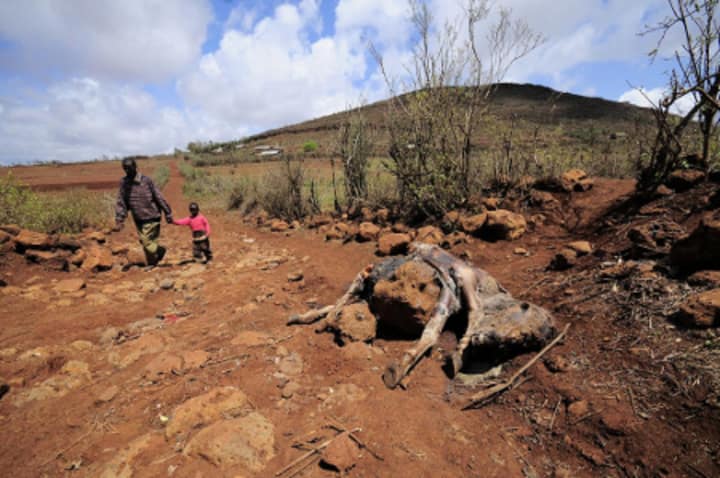In this photograph, under a vibrant blue sky dotted with puffy cumulus clouds, a barren, clay-like landscape stretches out. A mound approximately 30 feet high extends from the right edge to about three-quarters of the way across the image. In the foreground, an adult man in a purplish shirt and beige baggy pants is holding the hand of a young child dressed in a pink shirt and darker pants. They walk along a rough, red-hued dirt path scattered with rocks. Sparse, stunted foliage and leafless trees dot the area, hinting at a desert or mesa environment. The child appears to be around 2-3 years old, while the man seems to be rushing past a focal point of morbid curiosity—a decomposed carcass, possibly that of a baby bison, with legs and hooves still visible, draped over rocks and partially covered with dirt. The child glances at the remains as they walk forward.